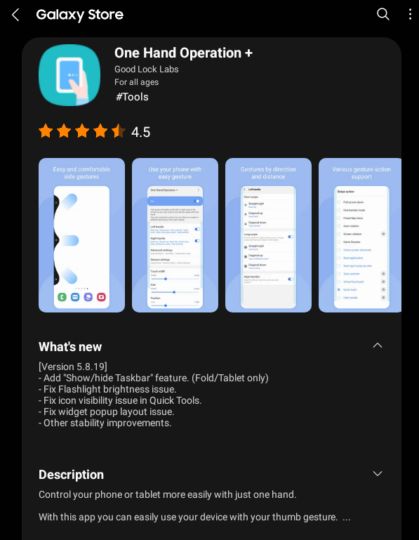Here is a cleaned-up and detailed caption for the provided image:

---

The image showcases the application "One Hand Operations Plus" available on the Galaxy Store. The app is developed under the branding "Good Lock Labs" and is suitable for users of all ages. It is categorized under "Tools" and boasts an impressive 4.5-star rating.

Displayed are four images that provide additional insights into the application's features, though the text within them is too small to decipher. 

The app version highlighted is 5.8.19, which introduces several updates and improvements:
- New feature: Show hidden taskbar (exclusive to foldable and tablet devices)
- Resolved issues with flashlight brightness
- Enhanced icon visibility in quick tools
- Fixed widget pop-up layout
- Various other stability improvements

In the "Description" section, the app promises to enhance the ease of controlling your phone or tablet with one hand, enabling users to navigate their device effortlessly using thumb gestures.